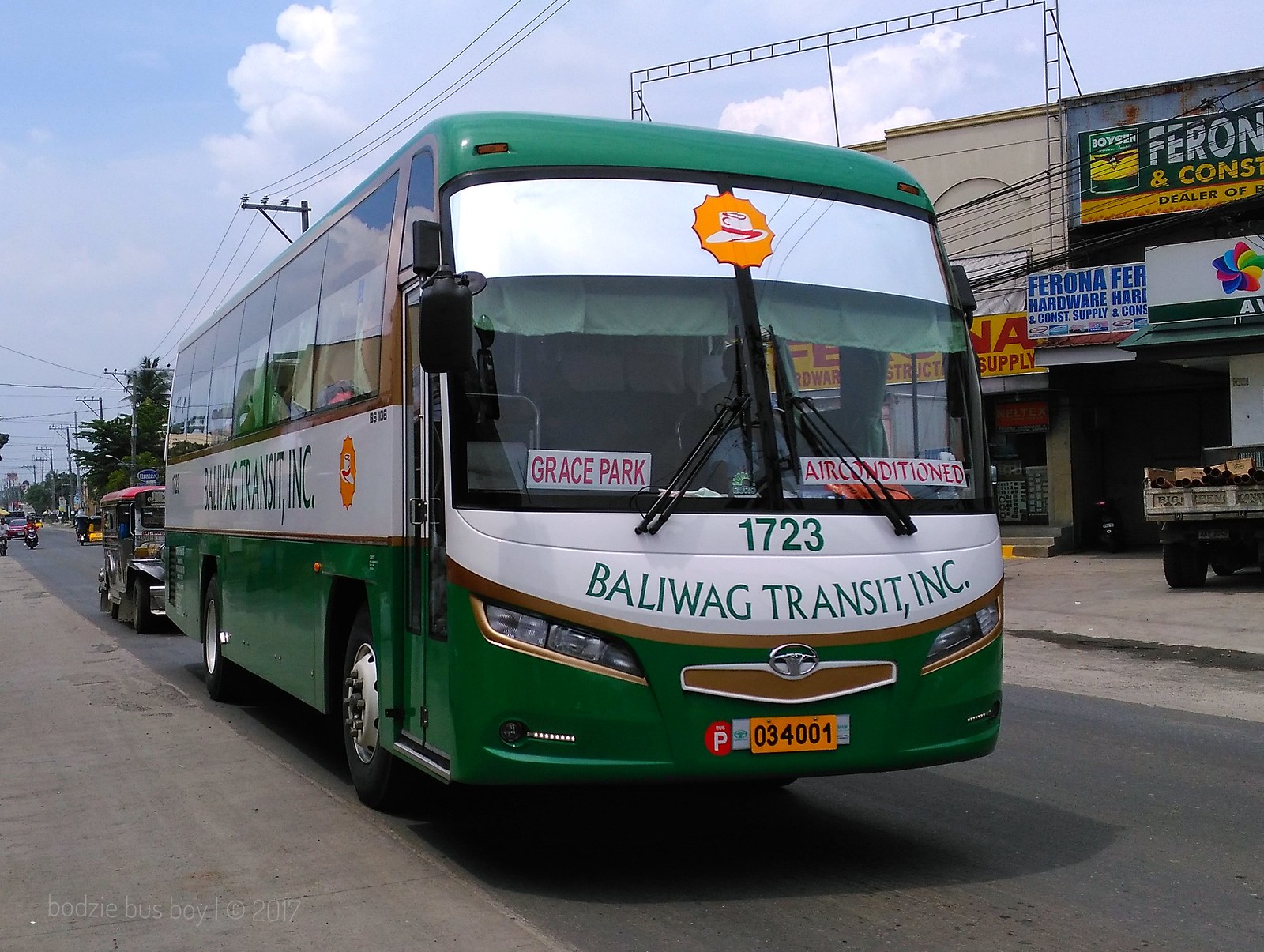The photograph, taken at street level on a bright day, features a passenger bus as its main focus. The bus, clearly labeled with the company name "Ballywag Transit Incorporated," is predominantly green with distinct white stripes down its side, including a white stripe above the front windows and a white panel below it. A green and white banner beneath the windows with the bus number "1723" and another sign that says "Grace Park Air Conditioned" can be seen. The bus also has a white banner over the driver's window featuring a logo of a hat in front of an orange spiky circle. The license plate, marked with the numbers "034001" on a yellow background, sits below the bus’s brown-trimmed front. It's parked along an urban street next to shops, one of which is identified as "Forona Hardware, Consta Supply." The scene includes some palm trees and telephone poles in the background, hinting at a possibly Asian location. The area appears to be lightly trafficked, with another vehicle, an old-style taxi or rickshaw, and motorcycles visible in the vicinity. Overall, the green, single-story bus with reflective windows suggests a vehicle used for tourist transport.